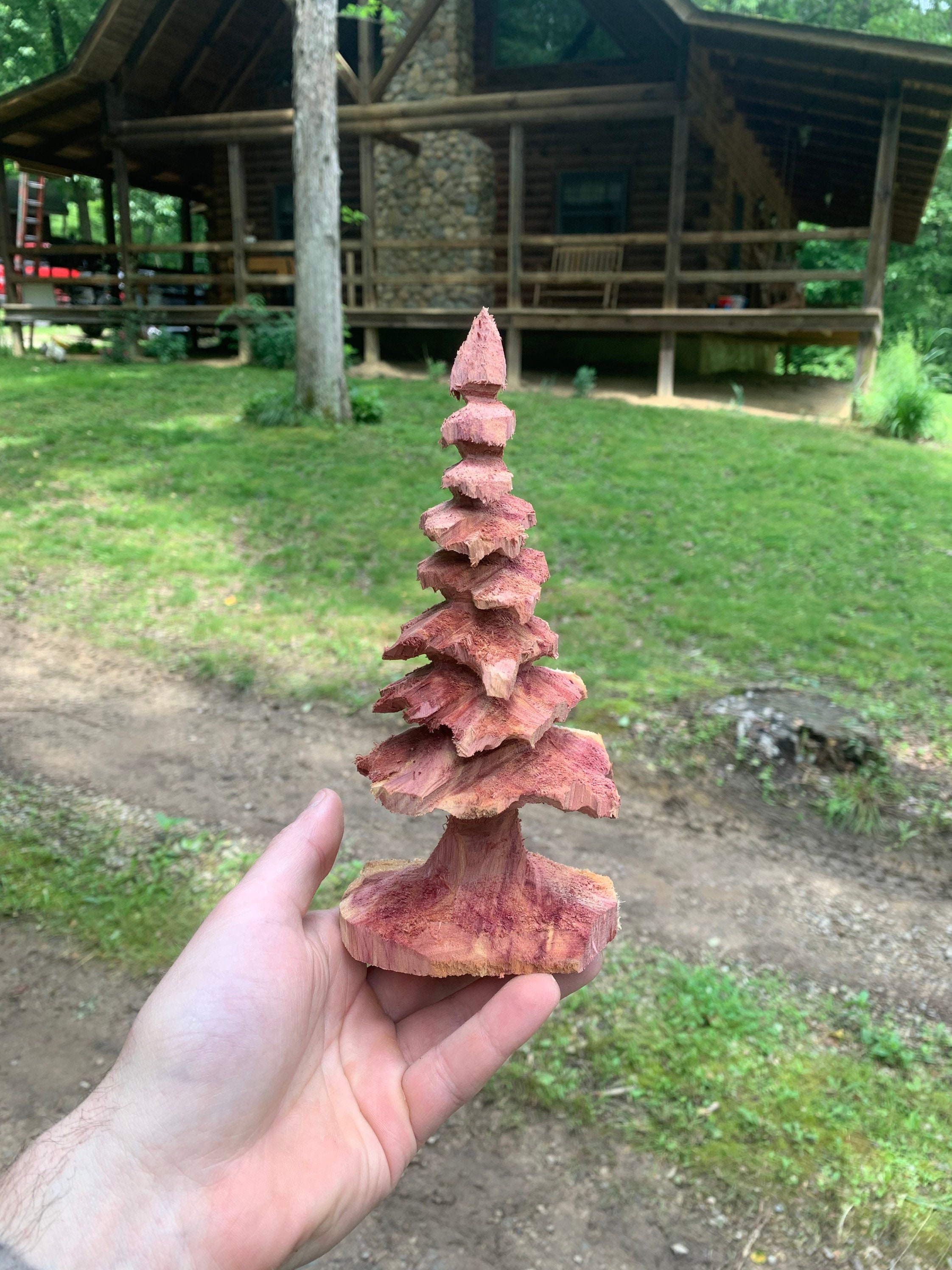In this somewhat aged photo taken outside at what appears to be a rustic summer camp, the main focus is a hand, extending palm up from the lower left corner, belonging to a Caucasian person, possibly a child. The hand delicately holds a carved wooden statue of an evergreen tree, crafted from reddish-brown, perhaps cedar wood, complete with a circular base and increasingly smaller layers as it ascends to a sharp point. The background reveals a large, brown wooden cabin with a wraparound porch and a charming stone fireplace on its exterior. The cabin, possibly a central dining hall, features wooden railings and a wooden bench. The lawn in front of the cabin is green but marked by twin tire tracks or trails etched into the ground. A single tree trunk emerges from the lawn, and there are dirt marks visible in the lower third of the image, hinting at the rustic and active environment typical of a summer camp. The overall scene exudes a nostalgic, serene vibe, accentuated by the simple yet delightful wood carving held in the foreground.